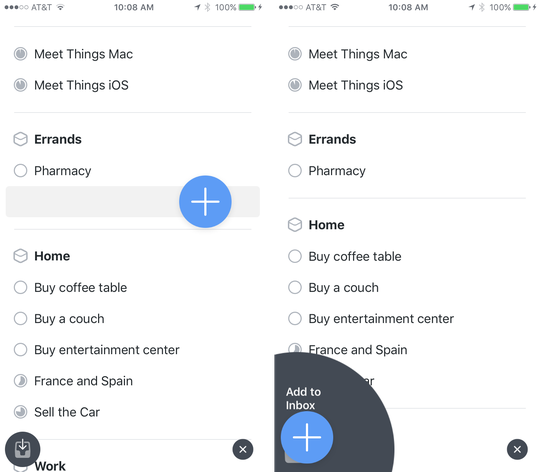The image showcases a user interface with two columns, each titled "MeetThings Mac" and "MeetThings iOS," both columns marked with check signs at the top. Each column contains a list of tasks: Errands, Pharmacy, Home, Buy Coffee Table, Buy a Couch, Buy Entertainment Center, France and Spain; however, "Sell the Car" is visible solely in the left column and partially obscured in the right column. At the bottom of the right column, there's a prominent gray quarter-circle with an embedded large blue circle featuring a white plus sign and the text "Add to Inbox." Similarly, beneath the "Pharmacy" task in the left column, there's an identical blue circle with a plus sign and an input space for typing.